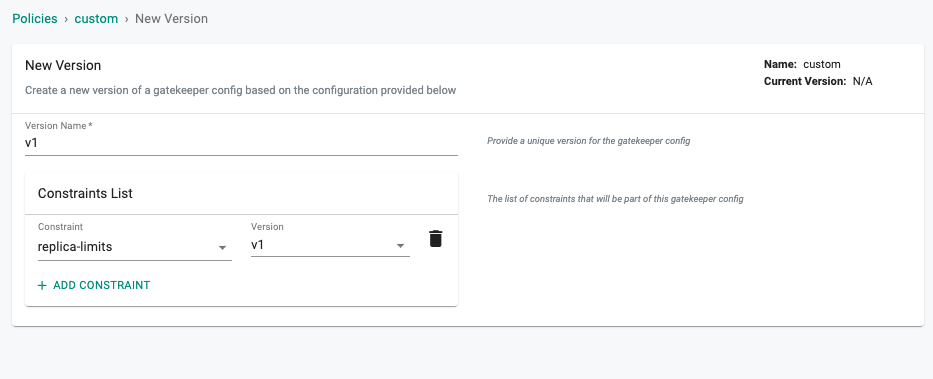The image is a screenshot of a webpage displaying a section related to gatekeeper configurations. The interface is designed within a faint gray rectangle, containing a central white rectangle. At the top left corner of the gray rectangle, the hierarchical navigation is shown: "Policies" (in green), followed by an arrow pointing to "Custom" (also in green), and another arrow pointing to "New Version" (in gray).

Within the white rectangle, an instructional text reads, "Create a new version of a gatekeeper config based on the configuration provided below." Below this text, input fields are provided. The first field is labeled "Version Name" and has the value "V1." 

Further down is a section titled "Constraints List," which includes an entry labeled "replica-limits" with a version "V1". To the right of this constraint, a black trash can icon allows for deletion. Beneath this, a green button labeled "+ Add Constraint" permits the addition of new constraints.

On the right side of the interface, additional guidance is provided: sections labeled "Name," "Custom," and "Current Version." A note clarifies, "Provide a unique version for the gatekeeper config and the list of constraints that will be part of this gatekeeper config."